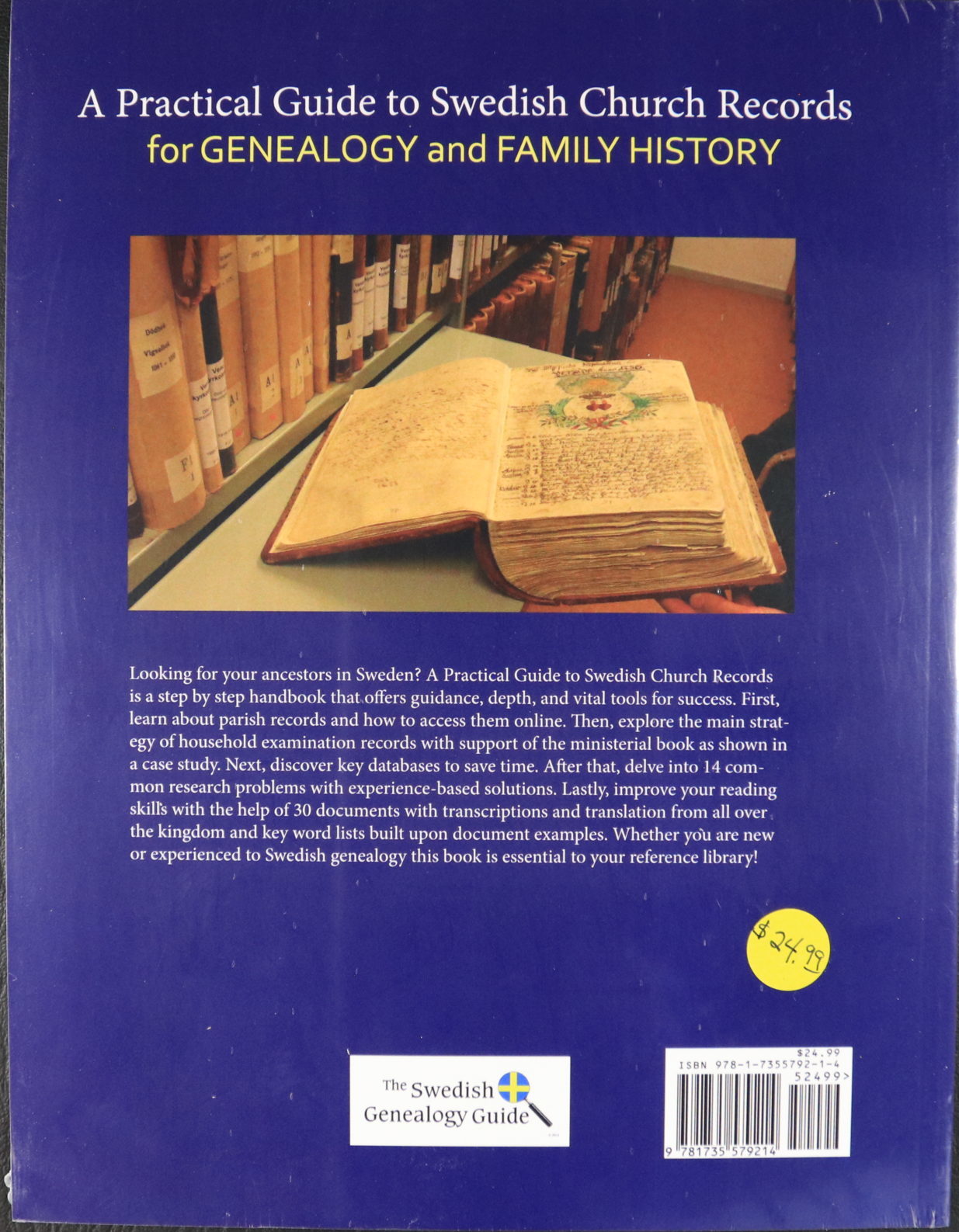The backside of this hardcover book features a blue background with white and yellow text. At the top, the white text reads, "A Practical Guide to Swedish Church Records," followed by yellow text that says, "For Genealogy and Family History." Below this, there is an image of an old, thick book with aged pages, possibly handwritten, lying open on a table, set against a backdrop that suggests a historical library scene with shelves of old book bindings.

Underneath the picture, there is a detailed description in white text: 

"Looking for Your Ancestors in Sweden? A Practical Guide to Swedish Church Records is a step-by-step handbook that offers guidance, depth, and vital tools for success. First, learn about parish records and how to access them online. Then explore the main strategy of household examination records with the support of the ministerial book, as shown in a case study. Next, discover key databases to save time. After that, delve into 14 common research problems with experience-based solutions. Lastly, improve your reading skills with the help of 30 documents with transcriptions and translations from all over the kingdom and keyword lists built upon document examples. Whether you are new or experienced in Swedish genealogy, this book is essential to your reference library."

At the bottom right corner, there is a yellow price tag marked $24.99 and a barcode. To the left of the barcode, within a small white rectangle, is the logo of "The Swedish Genealogy Guide," featuring a magnifying glass with the Swedish flag inside.